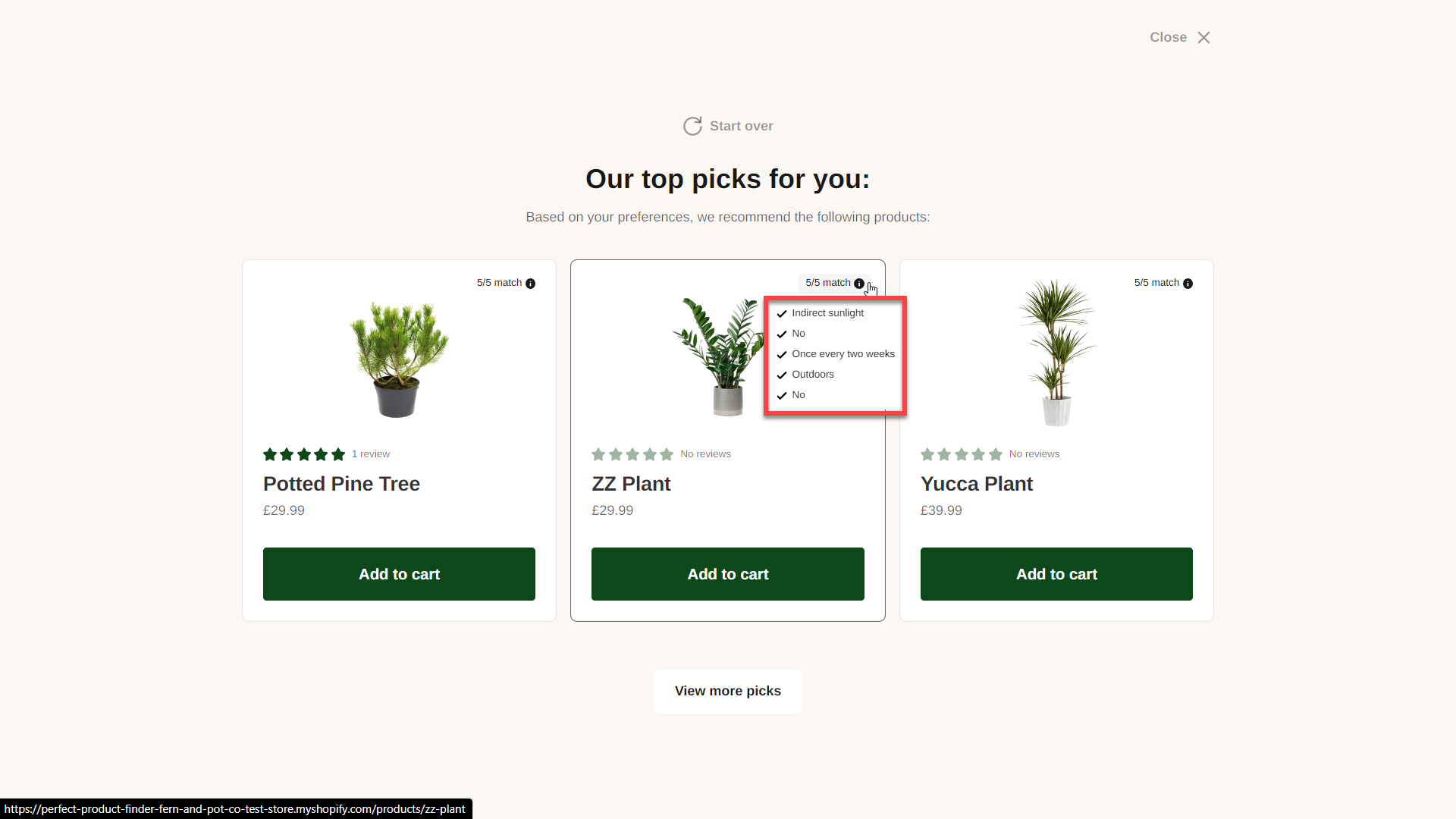A website features a product selection against an eggshell white backdrop. In the upper left corner, there is a white circle with the word "Close" and an "X" in black. Centrally at the top, a black refresh arrow icon is accompanied by the phrase "Start Over." Below, bold black text reads "Our Top Picks For You," followed by a smaller line: "Based on your preferences, we recommend the following products."

The section showcases three white boxes with featured plant products. 

**Left Product Box:**
- Image: A dark gray pot with a small bush.
- Rating: Five green, filled-in stars.
- Description: "Potted Pine Tree"
- Price: £29.99
- Action Button: A green bar with "Add to Cart" in white.

**Center Product Box:**
- Image: A gray pot with fern-like leaves.
- Features: Within a red-bordered box, it lists:
  - ✅ Indirect sunlight
  - ✅ Unreadable item
  - ✅ Once every few weeks
  - ✅ Suitable as outdoors
  - ✅ Unreadable item
- Rating: Five unfilled, dull green stars.
- Description: "ZZ Plant"
- Price: £29.99
- Action Button: A green bar with "Add to Cart" in white.

**Right Product Box:**
- Image: A white pot with three different height plants, resembling yucca plants.
- Rating: Five unfilled, dull green stars.
- Description: "Yucca Plant"
- Price: £39.99
- Action Button: A green bar with "Add to Cart" in white.